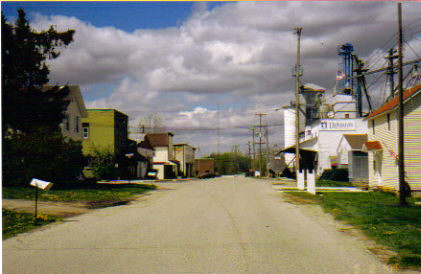This photograph captures a daytime view of a small town's road, composed of light gray asphalt marred by various cracks. The sky above is a blend of light blue and dark gray interspersed with large, billowy white clouds, creating a sense of layered overcast weather. The scene is flanked by buildings on both sides, mostly houses identifiable by their mailboxes. On the bottom left, a black pole supports a heavily angled white mailbox, hinting at a nearby dirt driveway. Further down the left side of the street, patches of green grass are visible, along with a dark green, almost black tree casting shadows near a house. The right side showcases a light tan or yellow house with a slanted red roof and a red portico, transitioning into a white factory marked by a tall blue crane and a cluster of telephone poles and wires. In the background, a white silo, additional telephone poles, and older style buildings add depth to the scene. The photograph is rich in detail, capturing the intersection of rustic residential charm and subtle industrial elements.